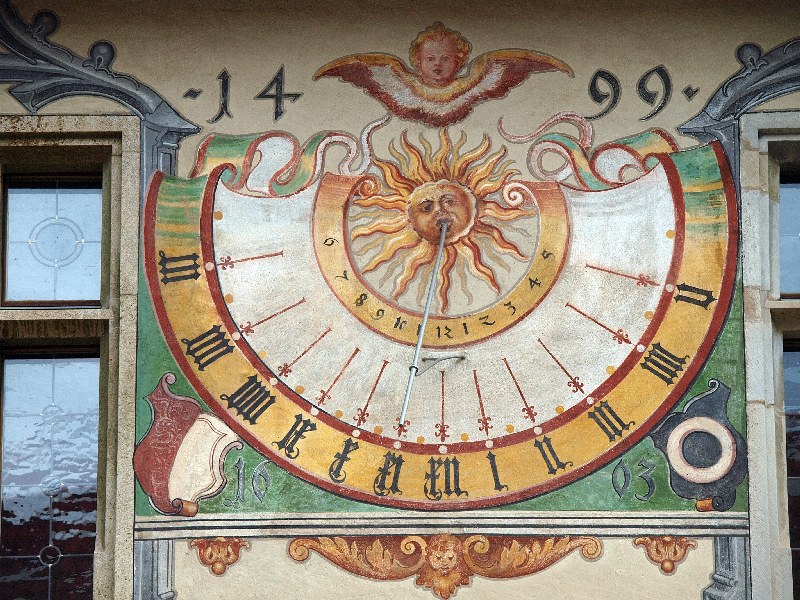The image showcases a building with a prominent concrete wall, featuring two large windows. Each window has a distinctive design, with panes intersected by two lines forming a cross within a circle. Positioned between the windows is a detailed painting. The painting includes a small mark labeled "14" on one side and "99" on the other. At the center of the artwork, an angelic face with wings is depicted in shades of yellow, white, and red. 

Above the angelic figure, a radiant sun is illustrated, emitting rays in vibrant hues of orange and yellow. Below this, there is a semi-circular clock face in orange and yellow, marked with black numbers. The clock face is segmented, with red arrows pointing to Roman numerals around its perimeter. Notably, the clock hand appears to emerge from the mouth of the sun within the image.

Surrounding the central artwork, there are accents of green paint, adding a contrasting backdrop to the vivid central elements.